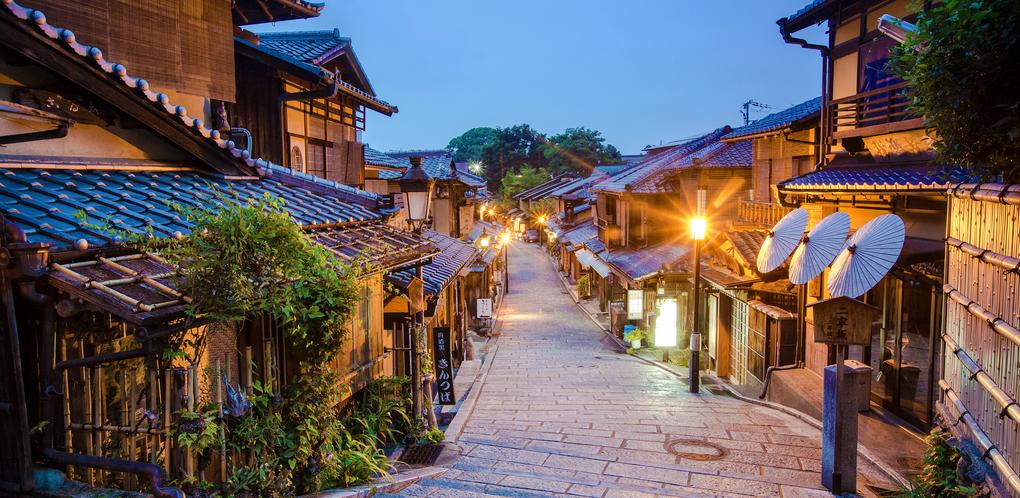A picturesque view down a charming village walkway, paved with neat brickwork. The sides of the walkway are lined with beautiful, attractive buildings that exude a quaint yet elegant vibe. The clear blue sky forms a stunning backdrop for the village scene. On the right side, there is a light pole and a building adorned with colorful umbrellas acting as awnings, featuring a higher level with a balcony and windows. This building is complemented by lush greenery. On the left side, an open-faced shop is also adorned with abundant greenery. All the buildings have a harmonious appearance with tan walls, brown trims, and edging, contributing to the village's symmetrical and clean aesthetic. Further down the walkway, light poles are illuminated, adding a warm glow to the scene, while trees in the background add to the village's natural charm.